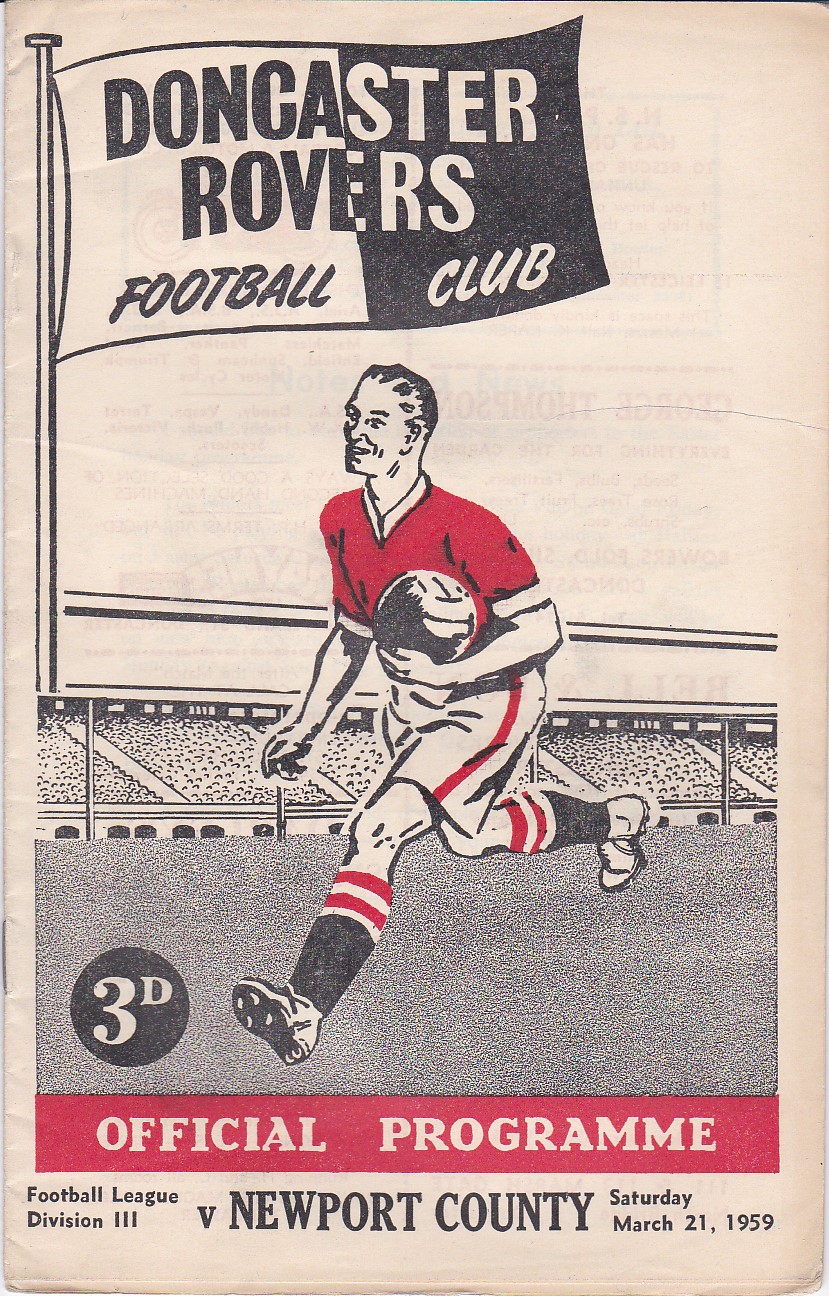The image depicts the front cover of an old and yellowed British football program from March 21, 1959. At the top left corner, an illustration of a divided flag reads "Doncaster Rovers Football Club" with its left side in white and right side in black. Below the flag, a graphic image of a footballer running with a ball clutched to his chest is central. He is depicted wearing a red jersey, white shorts with a red stripe down the side, and socks that are mostly black with two red stripes at the top. In the background, there's a detailed drawing of a football field and stands filled with the small heads of audience members. On the bottom left, within a black circle, it says "3D," and just above it in a red rectangular box, it reads "Official Programme." At the bottom of the cover, in black text, it states "Football League Division III v. Newport County, Saturday, March 21st, 1959." Overall, the primary colors of the cover are red, black, and white, though the paper has visibly yellowed over time.